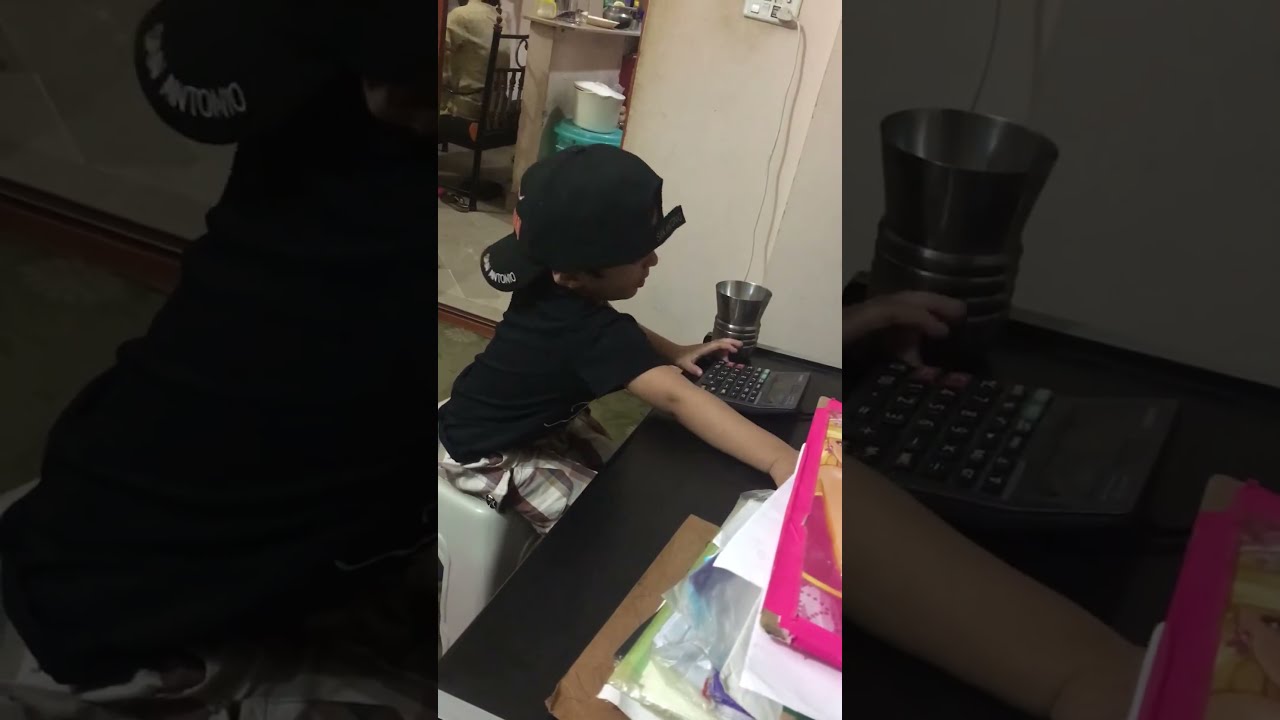The photograph is a horizontally rectangular image divided into three equal sections. The left and right sections are solid black, framing the central section which contains the photograph. This central area showcases a young boy, likely around three to five years old, with light brown skin. He wears an oversized black baseball cap turned backwards, with "San Antonio" printed in white on its adjustable strap. His attire includes a short-sleeved black t-shirt with unreadable white lettering and white, tan, and brown striped or plaid cargo shorts featuring square side pockets. The boy sits on a beige or gray plastic stool at a black desk, his hands resting on the surface before him. His left hand appears to be holding a small object that might be a remote control, while his right hand lies flat on the desk. To his left, there's a small stainless steel tin. The background reveals a white wall with some cords hanging down and a view into another room, which is somewhat cluttered. The floor features green patterned carpets. The boy's gaze is directed towards something on or beyond the desk, possibly a computer not visible in the image.